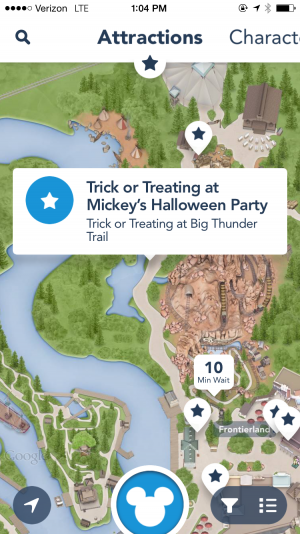This image appears to be a screenshot from a smartphone, displaying the interface of the phone at 1:04 p.m. The top-left corner indicates a Verizon LTE network connection, while the top-right corner shows the battery status and other icons. 

Below the status bar, the screen displays a section titled "Attractions" in bold, with a star symbol beneath it, suggesting it is part of a theme park navigation or guide app. The background features a detailed map depicting various themed areas, including water, green spaces, and brown pathways.

Centrally located on the screen is a white rectangle containing text about Halloween-themed activities: "Trick-or-treating at Mickey's Halloween Party" and "Trick-or-treating at Big Thunder Trail." 

At the very bottom center of the screen, a blue circle featuring a white Mickey Mouse icon, characterized by a large circle for the head and two smaller circles for the ears, can be seen.

This screenshot likely relates to a guide for Halloween festivities within a Disney theme park, highlighting specific trick-or-treat activities and locations.